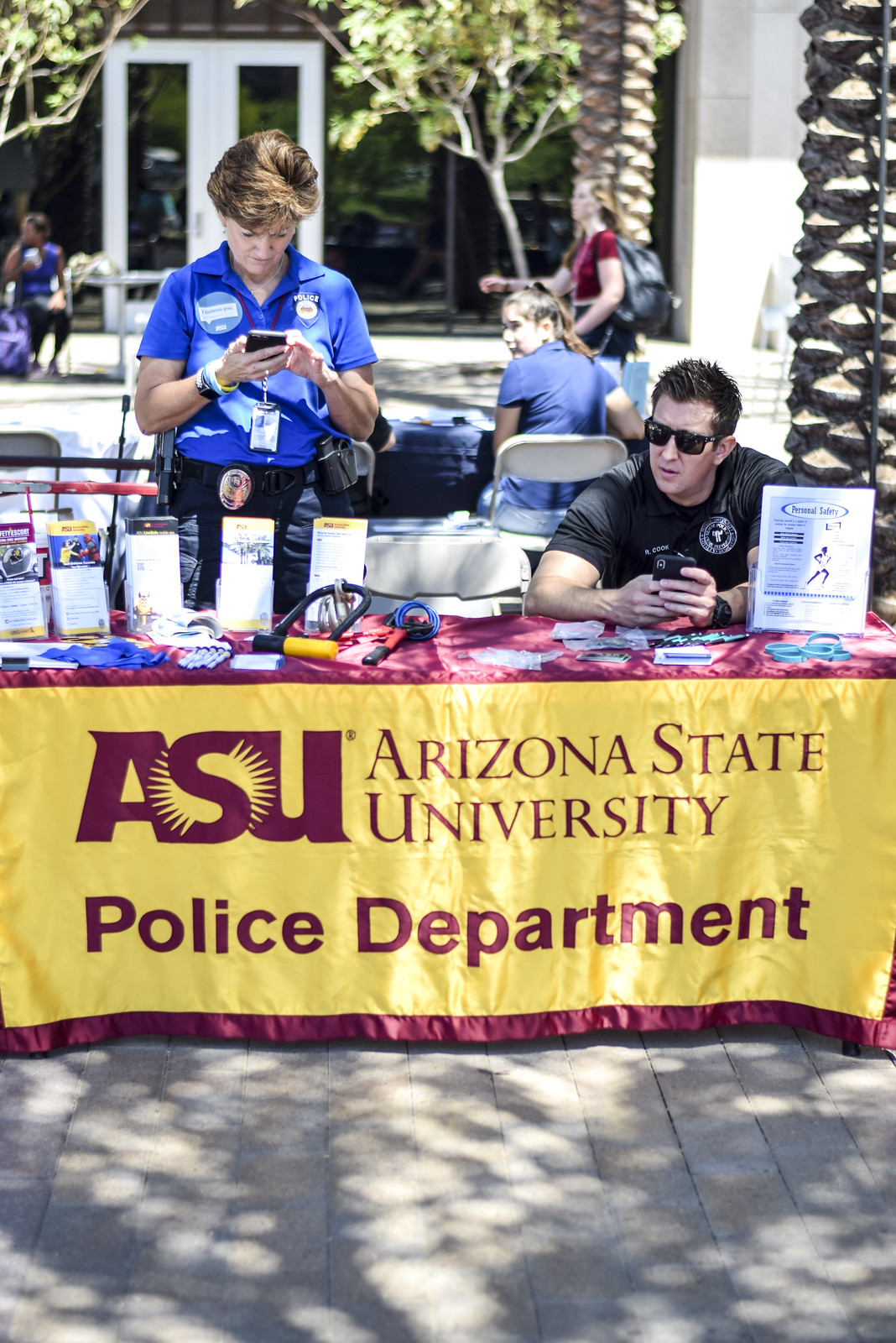This photorealistic image captures an outdoor booth setup at Arizona State University, identifiable by the red and yellow tablecloth adorned with "ASU Arizona State University Police Department" in red font. At the booth, a man with black hair, donning a black shirt and sunglasses, sits on the right side of the table, focused on his phone resting on the table. On the left side, a woman with short brown hair stands behind the table, wearing a blue shirt covered in numerous stickers, a lanyard, and dark blue or black pants, absorbed in her phone. The table is cluttered with pamphlets, demonstration devices like bike locks, and various giveaways. The backdrop features the lower parts of palm trees, students scattered around—some seated, some walking—and a white building with large dark windows across a paved area of small square stones in front of the booth.